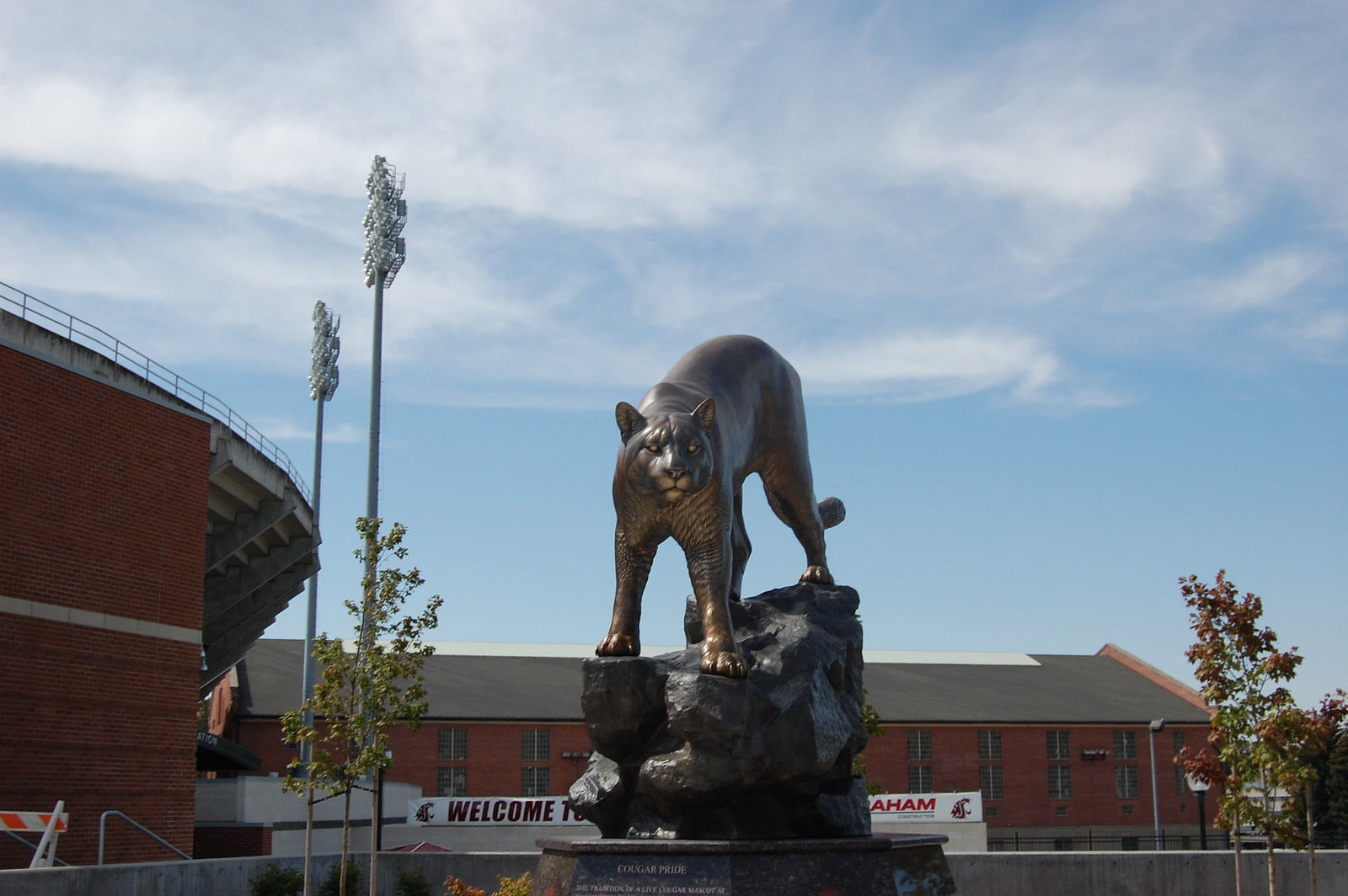In this vibrant photograph of a sunny day, the image captures the far end of a college field. Dominating the left-hand side, the back edge of a stadium is visible, showcasing tiered bleacher seating. The stadium's structure is a backdrop to the expansive, clear blue sky with only a few scattered white clouds, suggesting perfect weather.

At the very heart of the photograph stands a striking black lion statue, positioned boldly on a rock pedestal. The lion faces directly forward, commanding attention with its intense, yellowish eyes that contrast sharply with the dark hue of its body. Detailed sculpting highlights the intricate features of the lion's face, with a slightly less pronounced mouth that gives it a majestic yet fierce look.

In the background, behind the statue, a building can be seen, its facade adorned with several signs and lighting poles that add context to the setting, completing the scene of this collegiate environment.